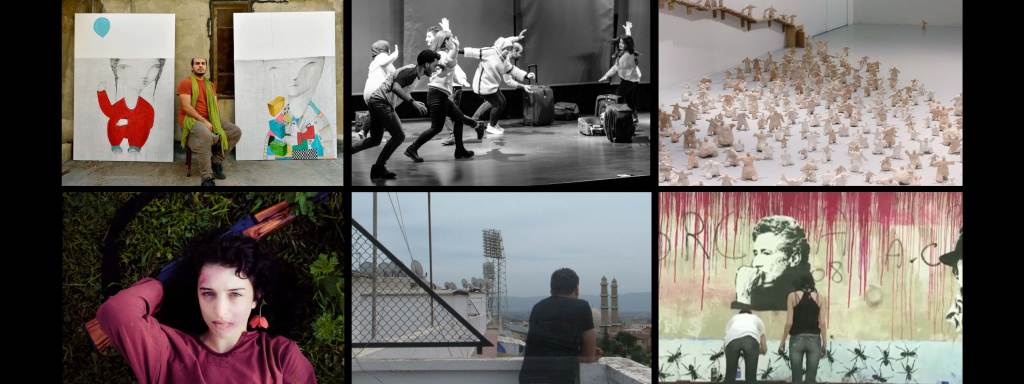In this detailed collage, we see six different images arranged in a vertical rectangle. Starting from the top left, there's a man wearing a red shirt sitting between two large canvases featuring his own artworks, characterized by figures with disproportionately large heads. The top center image is a black-and-white photo of people performing on a stage, with their arms flailing as they dance, and various travel bags scattered in front of them. The top right image shows a white room filled with numerous brown sculptures resembling fighting, war-like figures. 

Moving to the bottom row, the bottom left image is a close-up of a woman with black hair, wearing a burgundy long-sleeve shirt, lying on the grass with her right arm behind her head. She appears bruised around her mouth and forehead. The bottom center image features a man with black hair and a black shirt standing on a rooftop balcony, looking out over a cityscape with distinctly Asian architecture. A triangular gate frame can be seen on the railing to his left. The bottom right image depicts two people in front of a mural on a wall; the mural features ants painted along the bottom, portraits of people, various writings, and red paint dripping from the top.